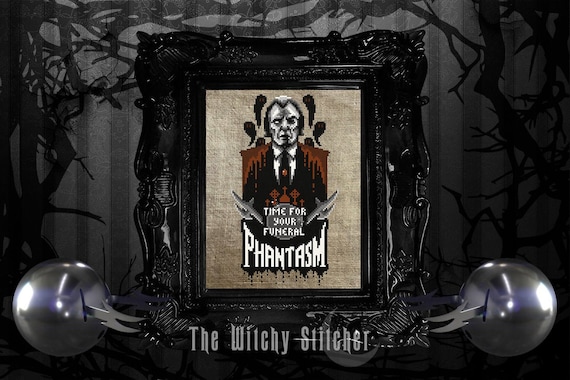The image depicts an intricately detailed gothic embroidery with a dark and eerie aesthetic. Dominating the center is an ornate black frame housing a pixelated, grim character reminiscent of a vampire. This figure is depicted in a black suit and tie, with red blood visibly running down from his shoulders. Supernatural elements surround his head, including ominous little ghosts with red eyes, enhancing the chilling atmosphere. The top text within the frame reads, "Time for your funeral," with the word "phantasm" underneath, styled in a dripping, black font.

The background of the piece is a haunting black and gray, featuring sharp, angular branches and shadowy motifs. At the bottom of the image, inscribed in gray text, is the phrase, "the witchy stitcher." Flanking this text are two translucent silver or gray balls with sharp knives or forks protruding outwards. This embroidery piece, filled with gothic charm and horror elements, appears perfectly tailored for fans of horror movies and gothic art.